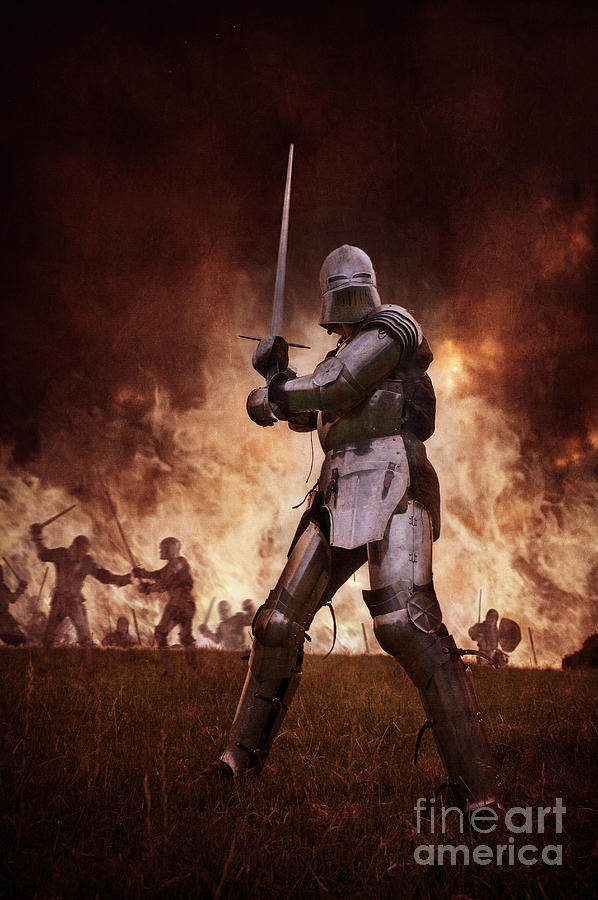The image is a detailed artwork portraying a dramatic medieval battlefield at night. Central to the composition is a prominent warrior clad in full armor, from helmet to leg guards, wielding a sword pointed upwards, suggesting he is either in attack mode or a defensive stance. Surrounding him is a chaotic scene with numerous other soldiers engaged in combat, their silhouetted figures adding to the sense of intensity. The battleground itself appears brown, likely due to the fire engulfing much of the space, which casts a diffused glow of orange, yellow, and hints of red. The night sky looms black above, enhancing the fiery contrast. The scene also includes patches of green grass on the ground, indicating a grassy field despite the destructive chaos. Notably, in the bottom right corner, the text "Fine Art America" is visible, marking the piece as a detailed and expressive interpretation of a medieval battle.